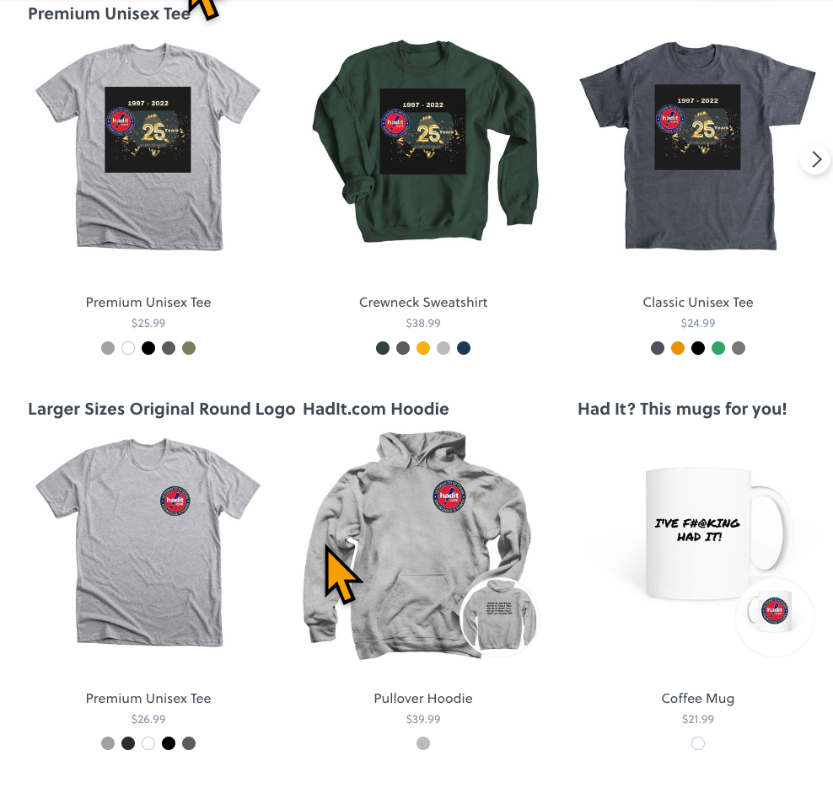This image from a retail website showcases a variety of premium unisex t-shirts, hoodies, and a coffee mug. At the top of the image, there are three t-shirts, with a yellow arrow pointing upwards to the text "Premium Unisex T." The first t-shirt is gray with a black square in the middle and the number "25" displayed prominently in the center. Below it is a green crewneck sweatshirt with long sleeves, also bearing the number "25" in black, priced between $19.97 and $20.22.

To the right of the crewneck, there is a classic unisex t-shirt priced at $24.99, featuring "25" in the center. This short-sleeve shirt is displayed alongside another premium unisex t-shirt, a gray short sleeve with the Hadit logo, which appears to depict a bat within a red circle.

Beneath these t-shirts, there is a hoodie with the original round logo of Hadit.com, available in larger sizes. This pullover hoodie is priced at $39.99 and has a small inset image showing the back, which contains some writing that is not legible in the image. An arrow points to the sleeve detail on the left side of the hoodie.

The display concludes with a coffee mug inscribed with “Hadit, this mug's for you. I've effing had it,” priced at $21.99. A small circular inset image shows the back of the mug for a comprehensive view.